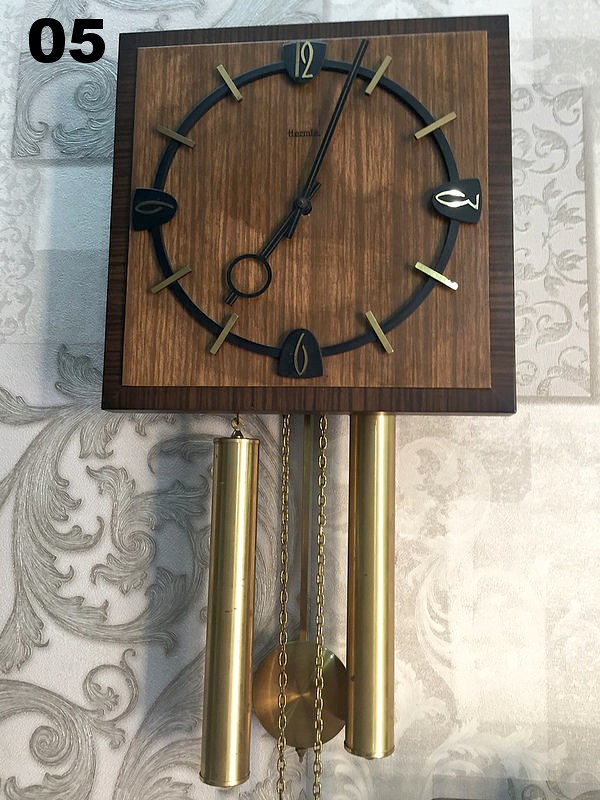This image features a beautifully crafted wall-mounted clock with intricate details. The clock, made predominantly of wood, showcases a square design with a dark border framing a lighter-toned wooden face, creating a striking contrast of various brown shades. The clock's hands are dark brown; the minute hand is notably long and currently sits between the 12 and 1 positions, while the shorter hour hand, distinguished by a small wooden circle near its tip, points between the 7 and 8 positions. The clock face includes the numerals 12, 3, 6, and 9, all rendered in a brass or gold color, with corresponding ticks for the remaining hours in the same metallic hue. Suspended from the bottom are two brass or gold-colored chains, both adorned with weighted pendulums, in addition to an actual pendulum, contributing to the clock’s classic and elegant aesthetic.